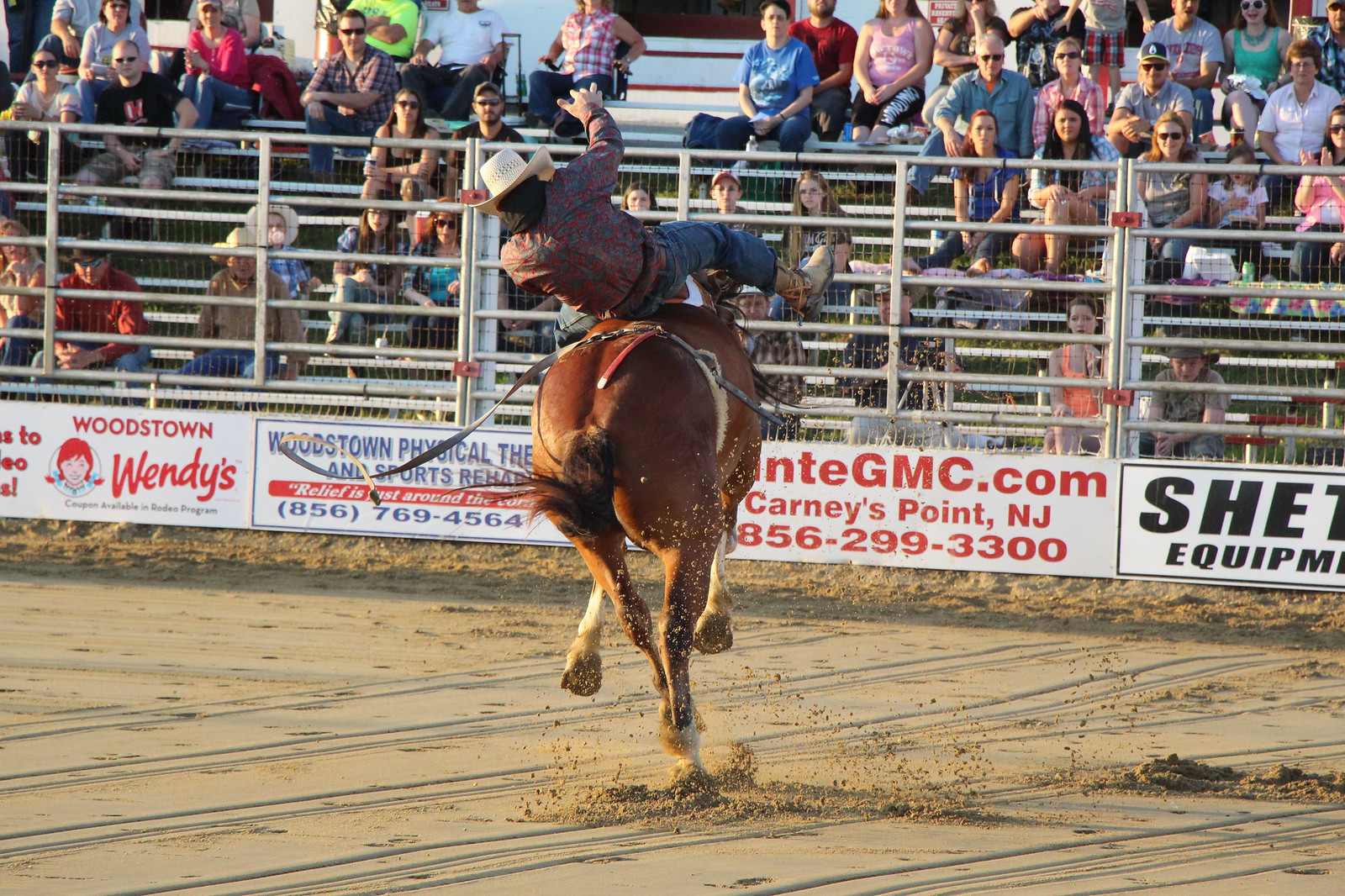The image vividly captures a thrilling moment at a rodeo event in broad daylight. Central to the picture is a powerful brown horse with its back end facing the viewer, its tail energetically bouncing as it kicks up dirt from the arena floor. Only one of the horse's hooves is touching the ground, emphasizing its dynamic motion. 

Mounted on the horse is a rodeo rider, clad in tan boots, blue jeans, and a stylish grayish-reddish long-sleeve shirt. He sports a cream-colored cowboy hat, and a black cloth is draped over his shoulders. The rider's right arm and leg are flung upward as he appears to be struggling to maintain his balance, leaning backward as though he's about to tumble off the horse. 

In the background, a grandstand filled with diverse spectators—men, women, and children, many of whom are wearing cowboy hats and sunglasses—captures the event's lively atmosphere. The bleachers are three-quarters full, with some attendees deeply focused on the rider's daring performance. 

At the bottom of the fence that separates the arena from the audience, several advertising posters are visible. These include sponsors such as Wendy's, Woodstone Physical, NTEGMC.com, Carnes Point, New Jersey, and a partly obscured equipment company. The presence of these signs adds a commercial backdrop to the rustic scene.